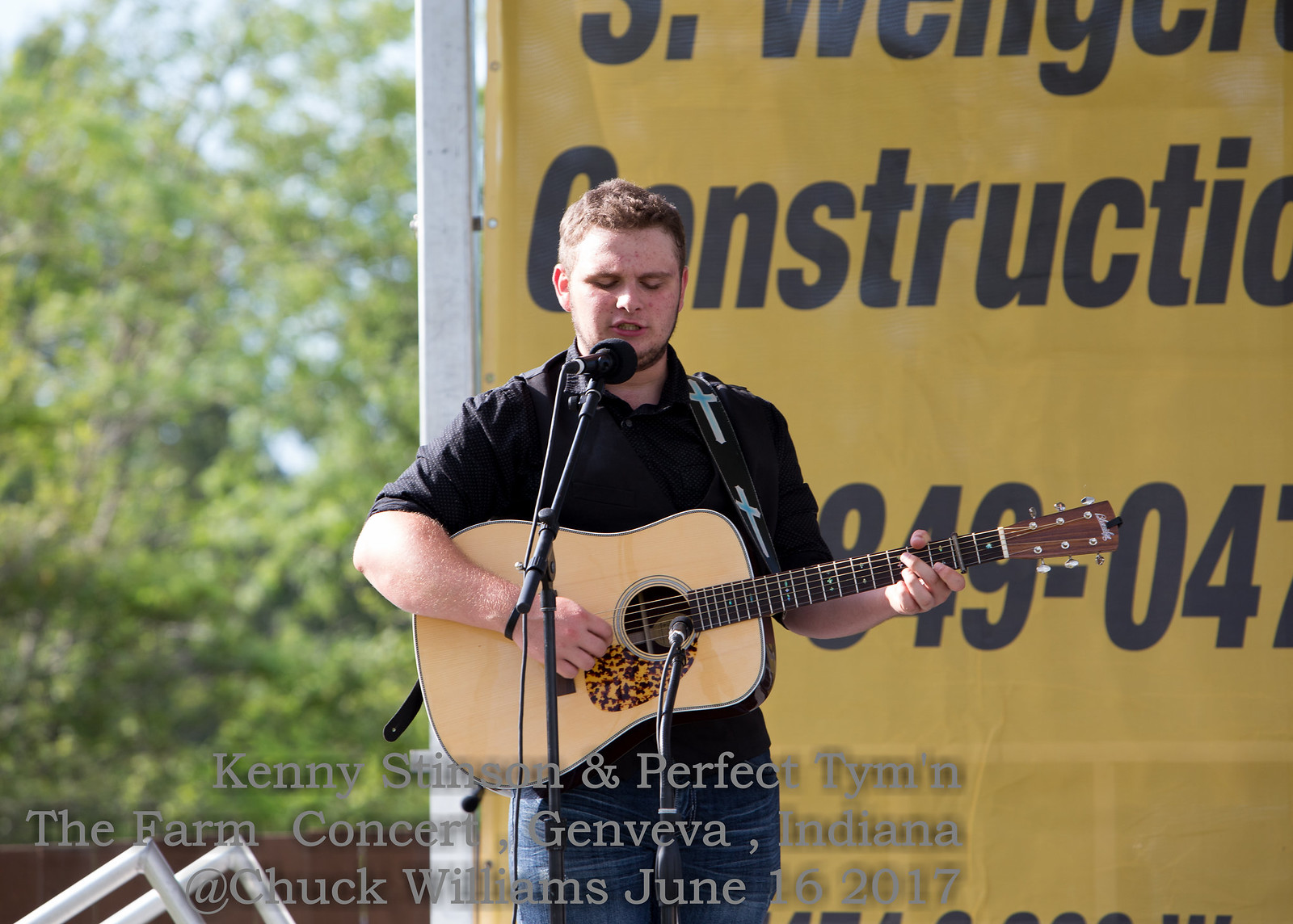An outdoor photograph captures a young white man with light brown hair and closed eyes, passionately singing into a microphone while playing an acoustic guitar. He is dressed in a collared black shirt and blue jeans, and around his neck, the guitar strap bears two Christian cross symbols, suggesting he might be performing Christian music. The guitar itself features a woodgrain finish with a leopard print design. Behind him, lush trees flank the left side, while on the right, a partially visible yellow sign reads "construction" and includes a phone number. Text at the bottom of the image reads, "Kenny Stinson & Perfect Tym’n, The Farm Concert, Geneva, Indiana, at Chuck Williams, June 16, 2017," indicating that Kenny Stinson is performing with the group Perfect Tym’n at this event. The photo was taken in rural Indiana on a sunny day, with the concert possibly sponsored by a construction firm.